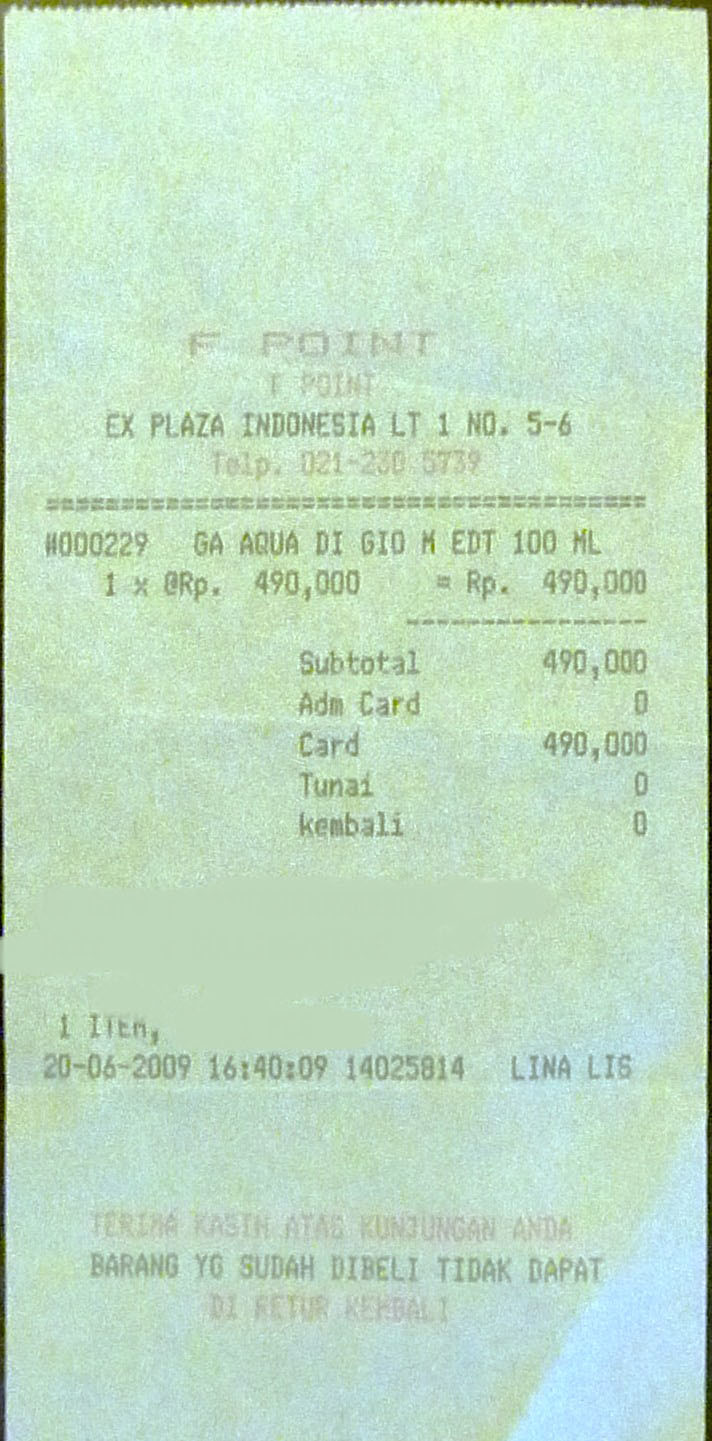The image shows a pale teal receipt with a combination of black and red printed text. At the top, it reads "F. X Plaza Indonesia LT 1, Number 5-6," followed by the telephone number "TEL 021-2386739." Below the contact information, two dashed lines underline the text, leading to details of the transaction. The receipt itemizes a purchase of 100 milliliters, likely a bottled item, costing 490,000 Indonesian Rupiah. The subtotal and card payment both indicate the amount of 490,000 Rupiah, with the word "Kembali" (Indonesian for "change") showing zero. The timestamp on the receipt is "6/20/2009 4:40 PM". Near the bottom, there is some additional text in Indonesian, including "Barang YG Sudah Dibeli Tidak Dapat," which translates to "Items that have been purchased cannot be returned."